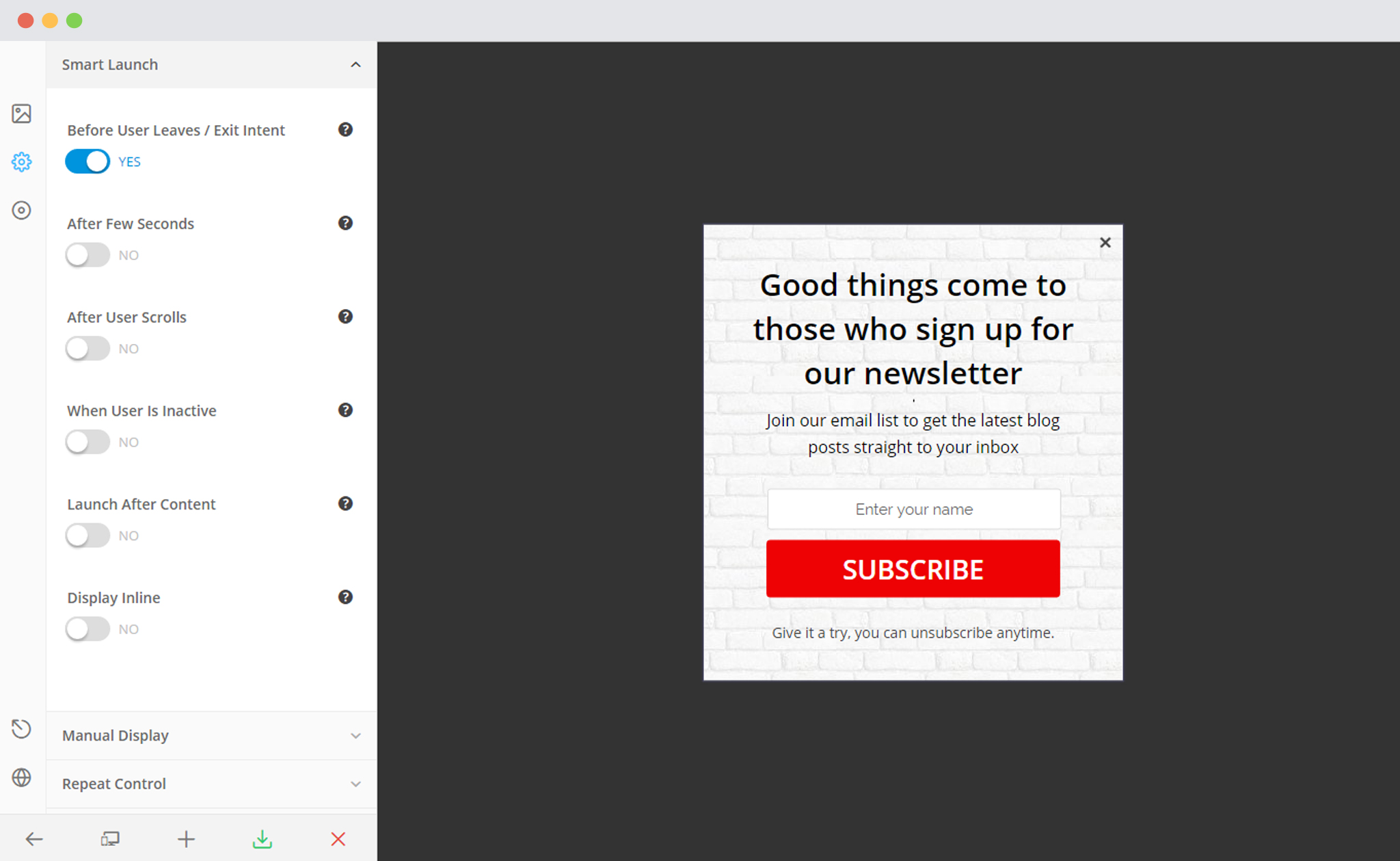Screenshot of a Mac computer screen displaying a pop-up window. The upper left corner features the familiar red, yellow, and green circles typical of Mac OS windows. The main section of the window has a header titled "Smart Launch." Below this, in gray text, it instructs "Before user leaves exit," and there is an option enabled by a button that says "Yes." Additionally, there are several operational instructions: "Hold for a few seconds, launch up content, manual display, repeat control," accompanied by small question mark icons for further clarification.

The lower half of the screen is occupied by another pop-up with a gray background. This section promotes newsletter sign-ups with the message: "Good things come to those who sign up for our newsletter. Join our email list to get the latest blog posts straight to your inbox." There is a field for users to enter their names and a prominent red "Subscribe" button. The entire layout is set against a background that mimics the appearance of white bricks.